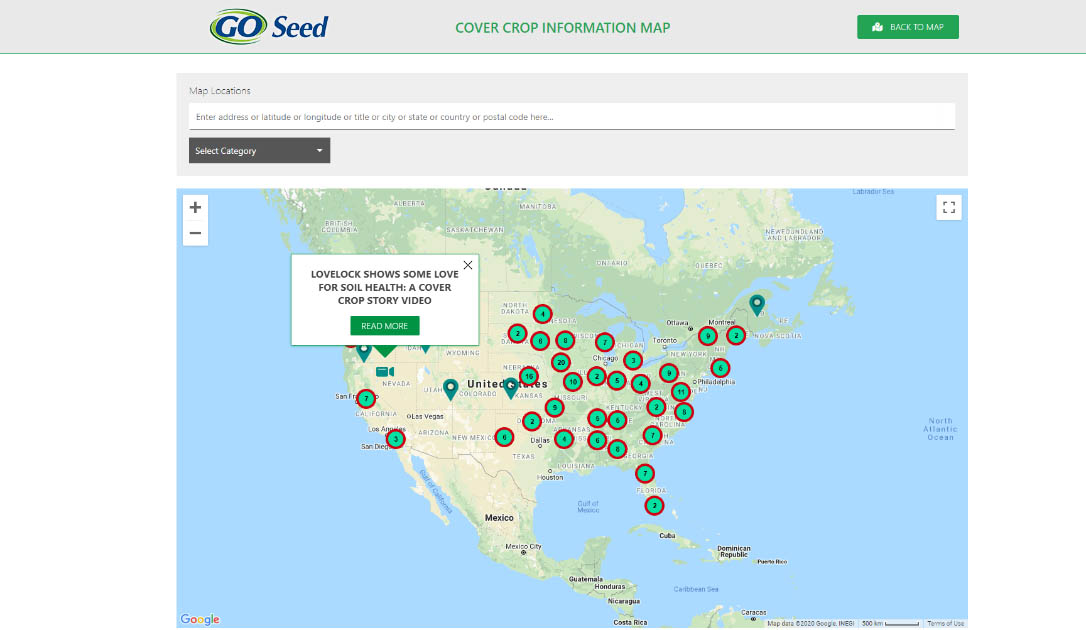This is a screenshot from the GoSeed website or application, prominently displaying a detailed map of the United States, with Mexico and Canada also partially visible. The main focus of the map is on the U.S., highlighting information related to crops and cover crops. 

The header features "GoSeed" in blue with a distinctive logo that includes a blue and green swirl around the word "Go." Below this, the text "Crop Cover Crop Information Map" is displayed in green. 

Underneath this title is a section labeled "Map Locations," featuring a search bar where users can enter an address, latitude, longitude, title, city, state, country, or postal code. Adjacent to the search bar is a drop-down menu for selecting specific categories.

The map itself is marked with numerous green circles, each surrounded by red circles with black numbers inside them, indicating various data points. One notable pop-up on the map is located over Nevada, featuring the text "Lovelock: Show Some Love for Soil Health – A Cover Crop Story Video," accompanied by a button labeled "Read More."

Overall, the map contains multiple numbered circles predominantly spread across the central and eastern United States, with a few located on the west coast. This interactive feature appears to allow users to click on the numbers to explore more detailed information about each location.